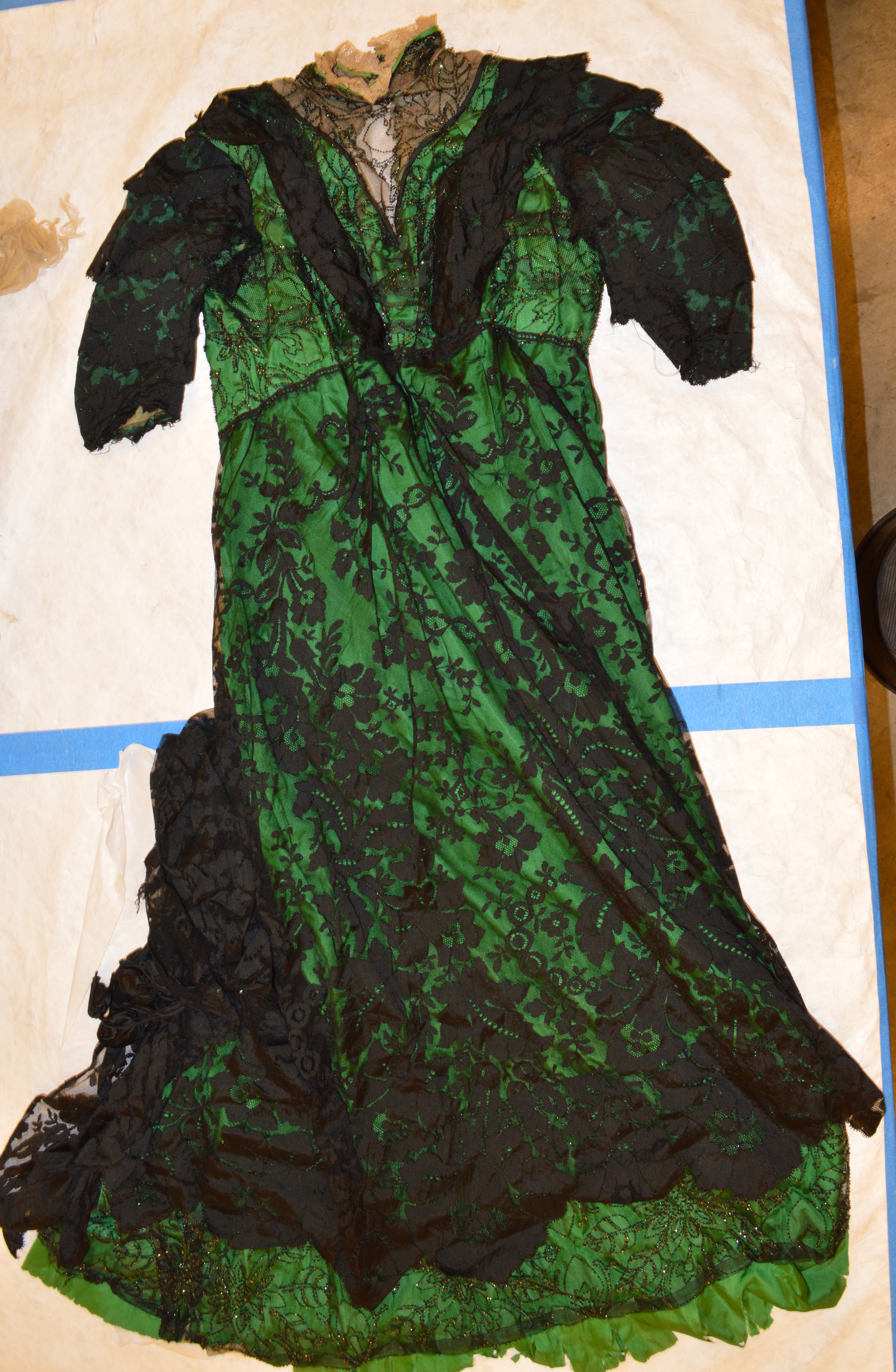This photograph features a vintage green dress, reminiscent of the iconic gown worn by Rose in the film *Titanic*, suggesting it might indeed be a similar or the same design. The dress is adorned with an intricate dark green lace overlay, adding to its antique charm. The collar stands out with its rich brown and gold detailing, giving it an elegant finish. The dress is carefully placed on white and blue parchment paper, enhancing its classic and timeless aura. The overall appearance of the dress evokes a sense of nostalgia, transporting viewers back to a bygone era.